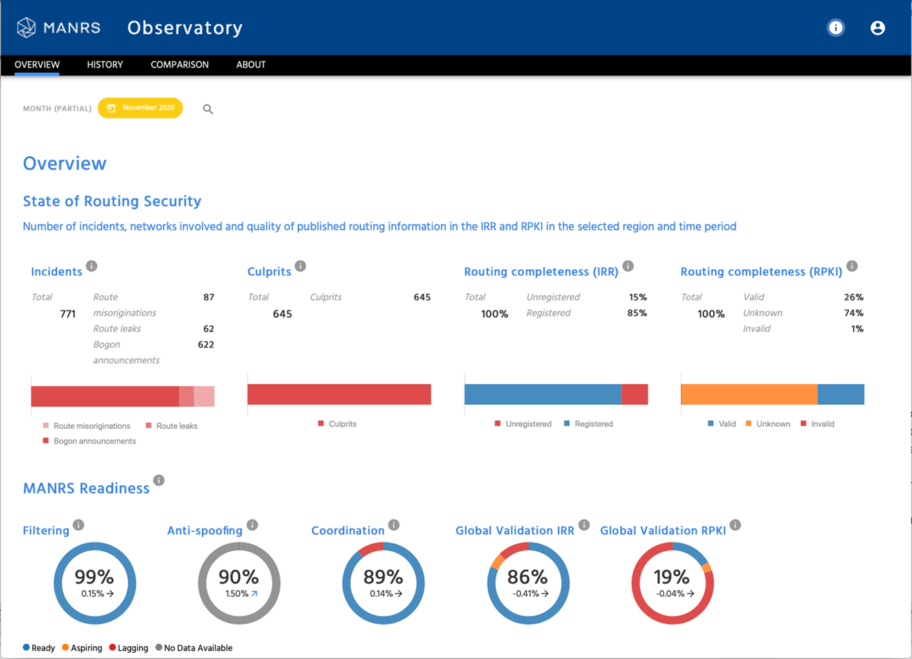The image is a horizontally rectangular screenshot of a webpage with a dark blue top border. On the upper left is the text "MANRS," followed by its logo, and in bold white letters next to it is "Observatory." Below this, there is a thin horizontal black banner displaying the navigation options: Overview, History, Comparison, and About. The "Overview" option is underlined in blue, indicating it is the current selection.

The main area of the screen has a white background with the heading "Overview" near the top. Underneath this, several subheadings are listed: "State of Routing Security," "Number of Incidents," "Networks Involved," and "Quality of Published Routing Information, IRR and RPKI" in the selected region and time period. 

Below these headings are four side-by-side bar graphs labeled with information corresponding to the subheadings: "Incidents," "Corporate Routing Completeness (IRR)," and "Routing Completeness (RPKI)." 

Further down the page is the heading "MANRS Readiness," under which there are three circles with various colors. Each circle displays a percentage at its center: Filtering at 99%, Anti-Spoofing at 90%, Coordination at 89%, Global Validation IRR at 86%, and Global Validation RPKI at 19%.